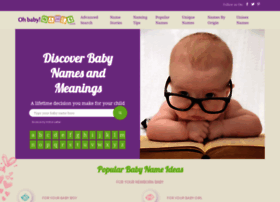The image captures a vibrant and engaging webpage dedicated to discovering baby names and their meanings. The headline, "Discover Baby Names and Meanings," is prominently displayed at the top of the page in white text against a deep purple background. Below this, a search box featuring a green magnifying glass invites users to explore further.

An adorable baby, wearing oversized black glasses, is the focal point of the image. The baby is lying on an open book or dictionary, adding a touch of charm and curiosity. Surrounding the baby, green letters are playfully scattered against the purple backdrop.

The webpage also highlights sections labeled "Popular Baby Names Ideas" in green text, indicating curated lists for users. At the very top, a banner with "Oh Baby" in purple text sets a welcoming tone. Various sections in purple text offer a structured layout for boys' and girls' names.

A purple bar at the top of the screen houses icons for social media platforms, suggesting users can easily connect and share content. Decorative elements, including pink floral designs, butterfly, and heart shapes, add a whimsical touch. The majority of the webpage features a beige background accented with purple and other vibrant colors, creating a visually appealing interface.

Overall, the baby with its striking glasses stands out, enhancing the playful and informative nature of this well-designed webpage.